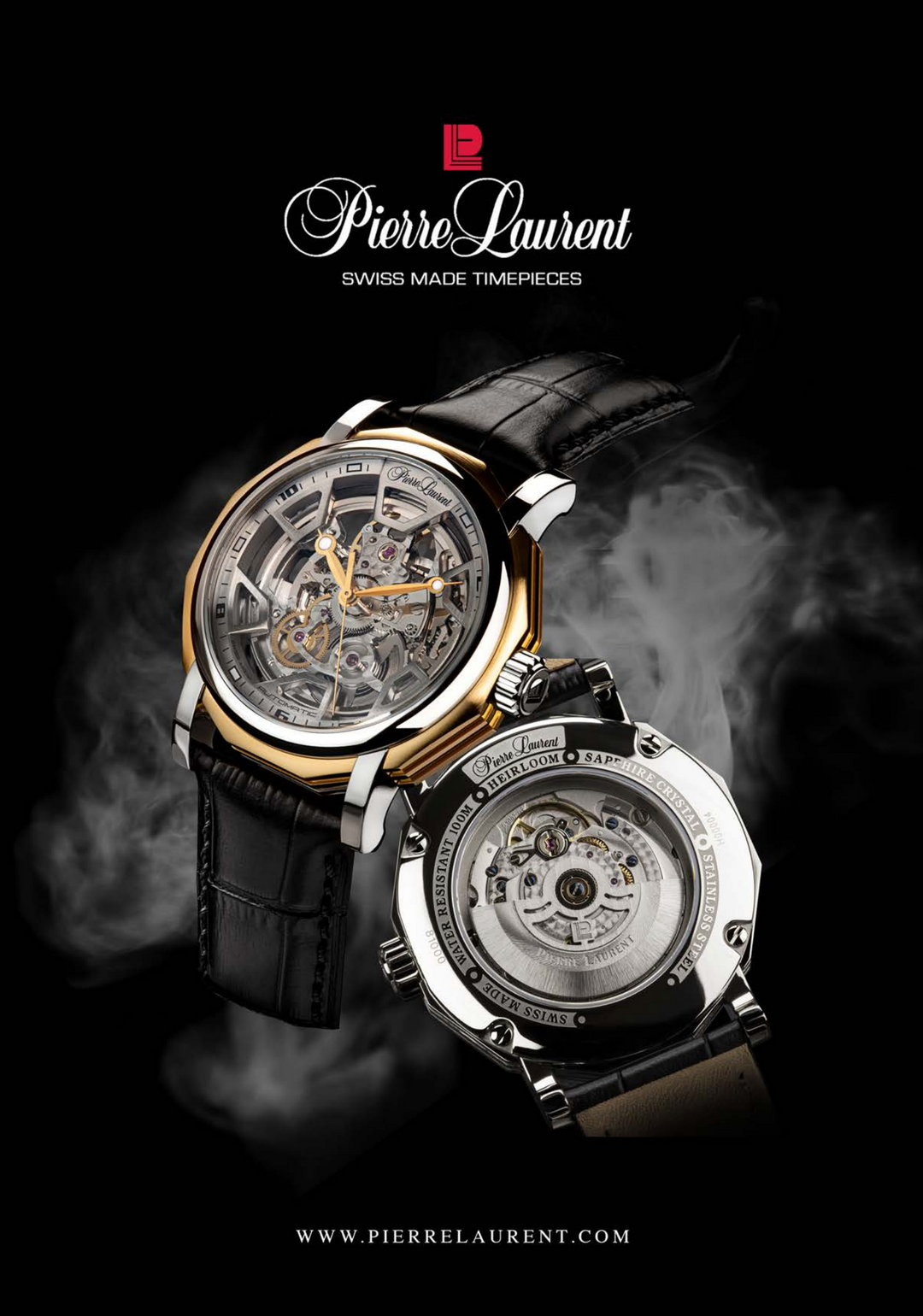This advertisement for the luxury watch brand Pierre Laurent, designed with a sleek black background, exudes sophistication suited for a high-end fashion magazine like GQ. Dominating the top of the ad is the distinctive red Pierre Laurent logo ("PL" with the P intricately connected to the vertical part of the L), and beneath it, “Pierre Laurent” is written in elegant white font, followed by “Swiss Made Timepieces.” Highlighted in the center are two exquisite watches, each showcasing impeccable craftsmanship and attention to detail. 

The watch on the left features a gold exterior and a meticulous design, allowing all the internal gears and springs to be seen through its transparent dial. Meanwhile, the watch on the right boasts a silver casing with similar transparency, revealing its intricate mechanical workings from the back window. Both timepieces are anchored against a light fog that softly enhances the overall aesthetic. Details such as the leather straps and the screws securing the design emphasize the high quality and precision. The high-resolution image concludes with the brand's website, www.pierrelaurent.com, discreetly positioned at the bottom, inviting viewers to explore more about Pierre Laurent’s luxurious offerings.